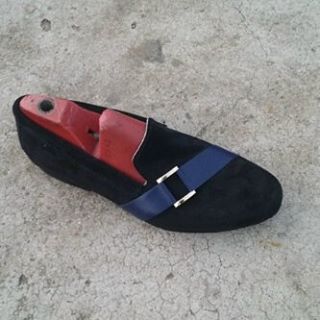The image features a black loafer-style sandal set against a gray concrete background. The shoe, possibly made of leather or suede, has a somewhat pointed toe and a wide navy blue ribbon running diagonally across its top. This ribbon is adorned with a chrome-colored decorative buckle, positioned towards the right side above where the pinky toe would be. Inside the shoe, there is a red shoe tree— a adjustable wooden form used to maintain the shoe's shape. The concrete surface is textured with visible cracks, adding a rugged contrast to the polished look of the loafer. There is also a drilled hole in the heel of the shoe.